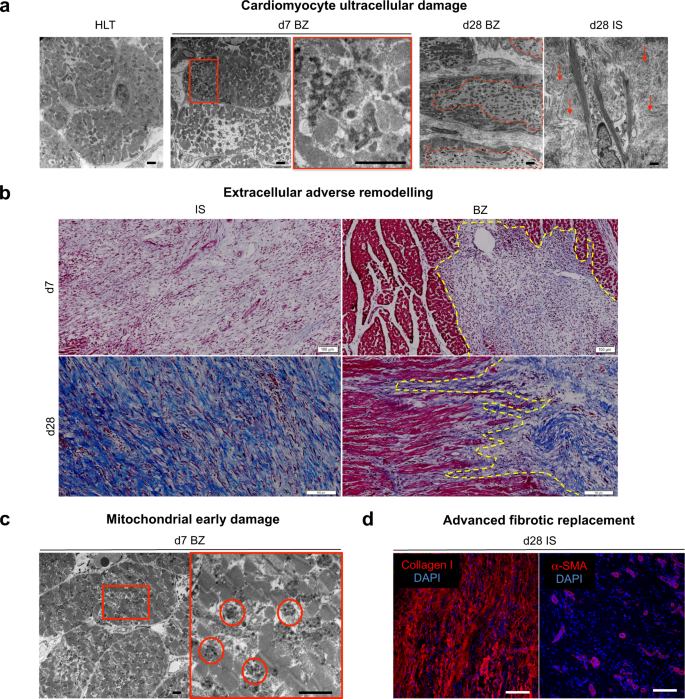The scientific medical image displays a detailed examination of cardiomyocytic ultracellular damage, categorized into four sections: A, B, C, and D, likely for educational purposes. 

Section A, labeled "Cardiomyocyte Ultracellular Damage," includes five grayscale images highlighting cellular damage with red boxes and arrows to indicate specific areas of adversity. 

Section B, titled "Extracellular Adverse Remodeling," features four colorful microscopic images in shades of blue, pink, and yellow, illustrating adverse changes outside the cells.

Section C, "Mitochondrial Early Damage," returns to grayscale imagery, marked by red boxes and circles to pinpoint areas of mitochondrial impairment.

Section D, "Advanced Fibrotic Replacement," presents images with a black background and hues of red, purple, and blue, indicative of advanced fibrotic changes within the tissue. 

Each section provides a visual representation of different stages of cellular and tissue damage, from mitochondrial impairment to fibrotic replacement.